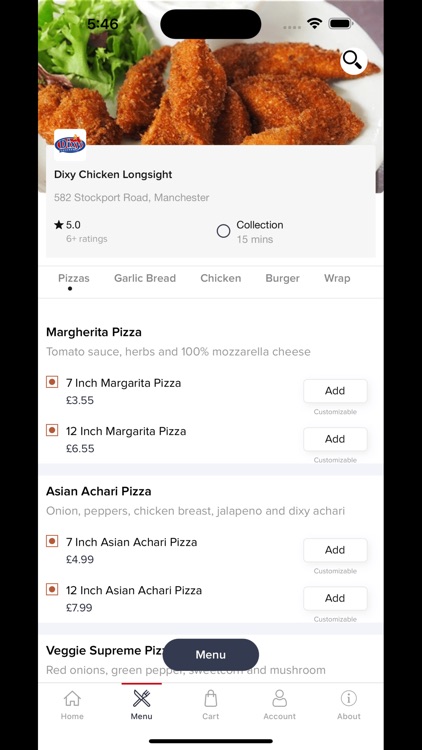The image is a screenshot of a digital menu from a restaurant. At the top, it features an image of fried chicken. Below the image, the text displays the restaurant name "Dixie Chicken Long Sight" and the address "582 Stockport Road, Manchester." It boasts a 5.0-star rating and indicates that a collection order will be ready in 15 minutes.

The menu appears to be focused on the "Pizzas" section. Listed items include:

1. **Margherita Pizza**:
   - **Description**: Made with tomato sauce, herbs, and 100% mozzarella cheese.
   - **Sizes and Prices**: 
     - 7-inch for $3.55
     - 12-inch for $6.55

2. **Asian Akari Pizza**:
   - **Description**: Topped with onion, peppers, chicken breast, jalapeno, and Dixie Akari.
   - **Sizes and Prices**:
     - 7-inch for $4.99
     - 12-inch for $7.99